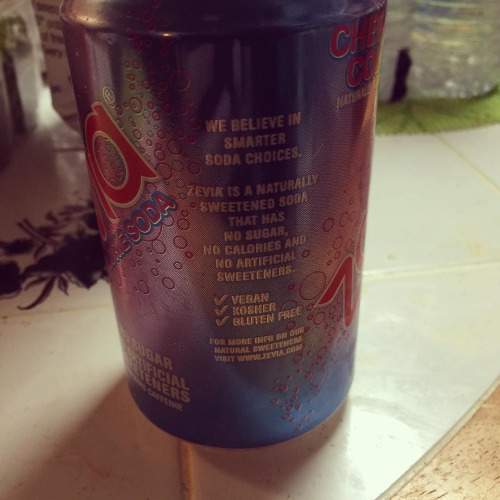In a dimly lit interior, a can of soda stands prominently against a background of white or off-white tiling. The can, captured at a slight angle, features a deep purple hue that fades into shades of blue and red. The design includes a light red background with red circular elements symbolizing bubbles. Written vertically in white text, the label reads, "We believe in smarter soda choices." Further details reveal that the soda, branded as "Zivia," is naturally sweetened and contains no sugar, no calories, and no artificial sweeteners. Additionally, the labels highlight its dietary benefits with checkmarks indicating that the beverage is vegan, kosher, and gluten-free. The top of the can is not visible in the photo.